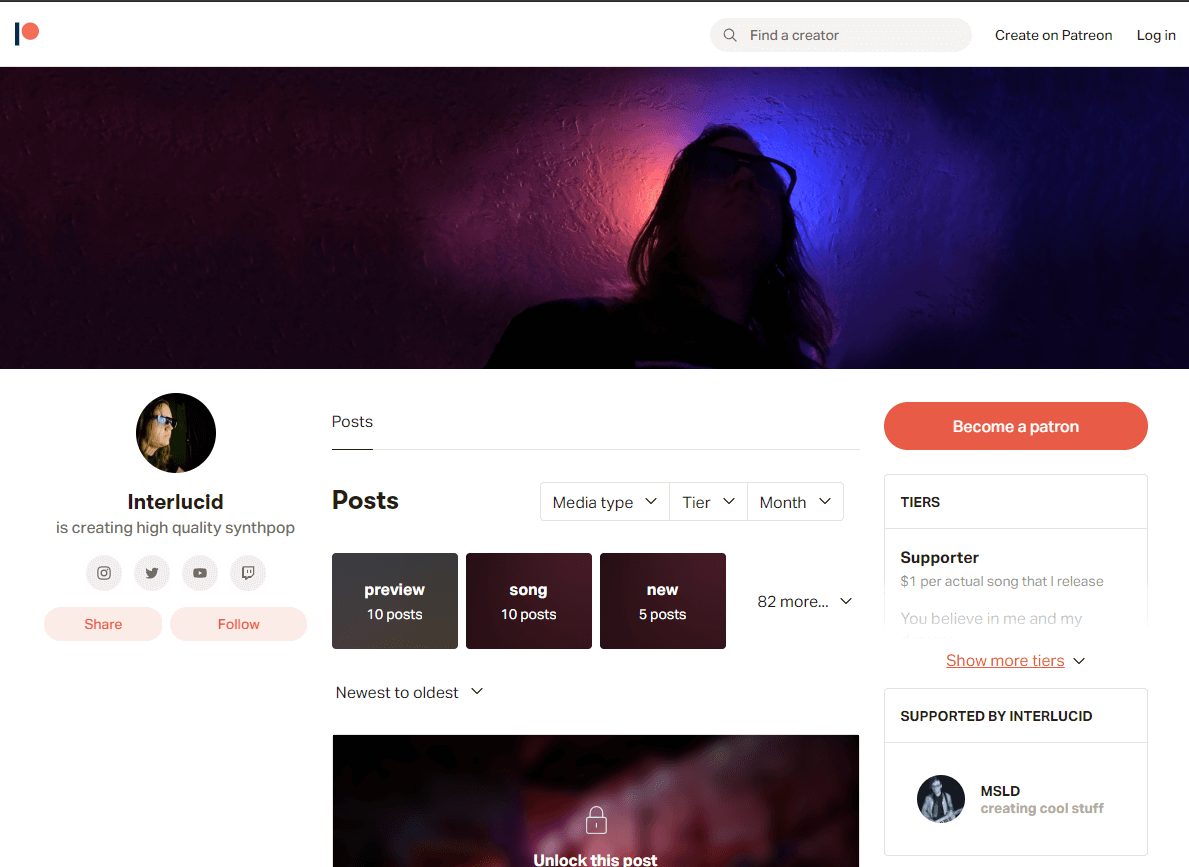This appears to be a page from the website Patreon featuring an artist named Interlucid. At the upper left corner, you can see a small vertical black line with a red circle next to it. Moving to the right, there's an oval search bar with a magnifying glass icon and the words "Find a creator" inside it. Next to the search bar, in dark letters, it says "Create on Patreon," followed by a "Login" button.

At the top section of the page, there is a graphic likely representing the person whose page this is—depicted as a silhouette of someone with long hair. Below this graphic, to the left, there is what seems to be the creator's icon or avatar: a round dark circle containing an image. Underneath this icon, the text reads "Interlucid is creating high-quality synth-pop."

Additionally, the page features a prominent red oval button that says "Become a patron." Other visible elements include various labels like "Post," "Me," "Type," "Tier," "Month," "Tier Supporter," "Supported by Interlucid," "PV Song," and "New." These likely pertain to different sections or features available to supporters or patrons on this page.